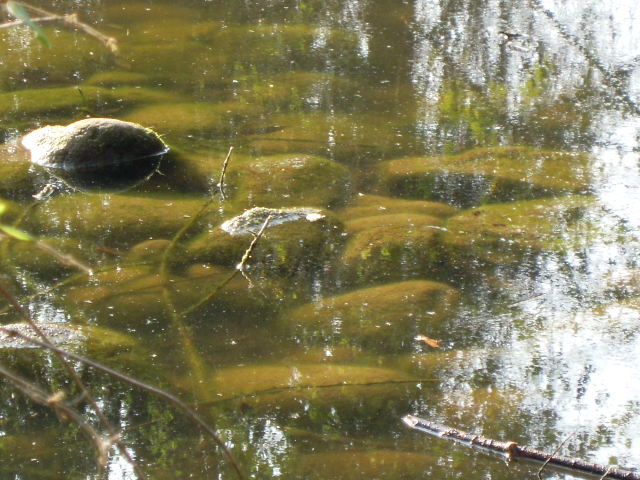This wide rectangular image captures a still, reflective body of water, possibly a lake or very slow-moving river, surrounded by nature. The water is adorned with stones, some of which are covered in algae and moss, indicating slow movement and tranquility. Small, furry-green objects resembling moss or algae float close to the water's surface, tinted with shades of greenish-brown and gray. Dominating the top left corner, a stick lies in the water among other scattered branches and limbs. Another stick or gray object pokes just above the surface. The right side of the image features a crystal-clear reflection of a light blue and white sky, framed by long-branched trees with green leaves. This setting appears to capture an outdoor scene on a semi-cloudy day, with the calmness of the water contrasting with the vibrant reflections of the sky and surrounding nature.